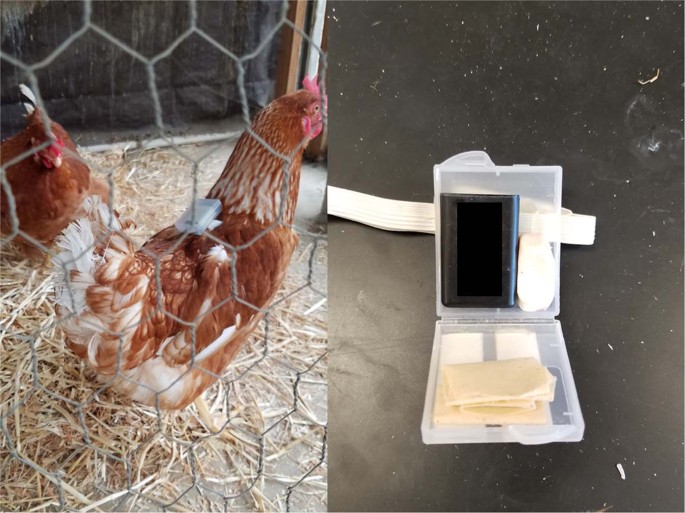This is a split-colored photograph taken outdoors, featuring two images side-by-side. The left image captures two brown chickens, possibly roosters, inside a wire-caged coop with straw covering the floor. The chicken in the foreground, which has red wattles and a crest, is standing in profile, revealing a clear plastic box strapped to its back with a white elastic band, resembling a small backpack. The chicken in the background is sitting quietly. The right image provides a close-up of the same clear plastic box, which is open like a clamshell and rests on a black surface. Inside the box, there are items including a black triangular object and a folded piece of paper, possibly indicating the box's purpose as an electronic tracking device for the chickens.